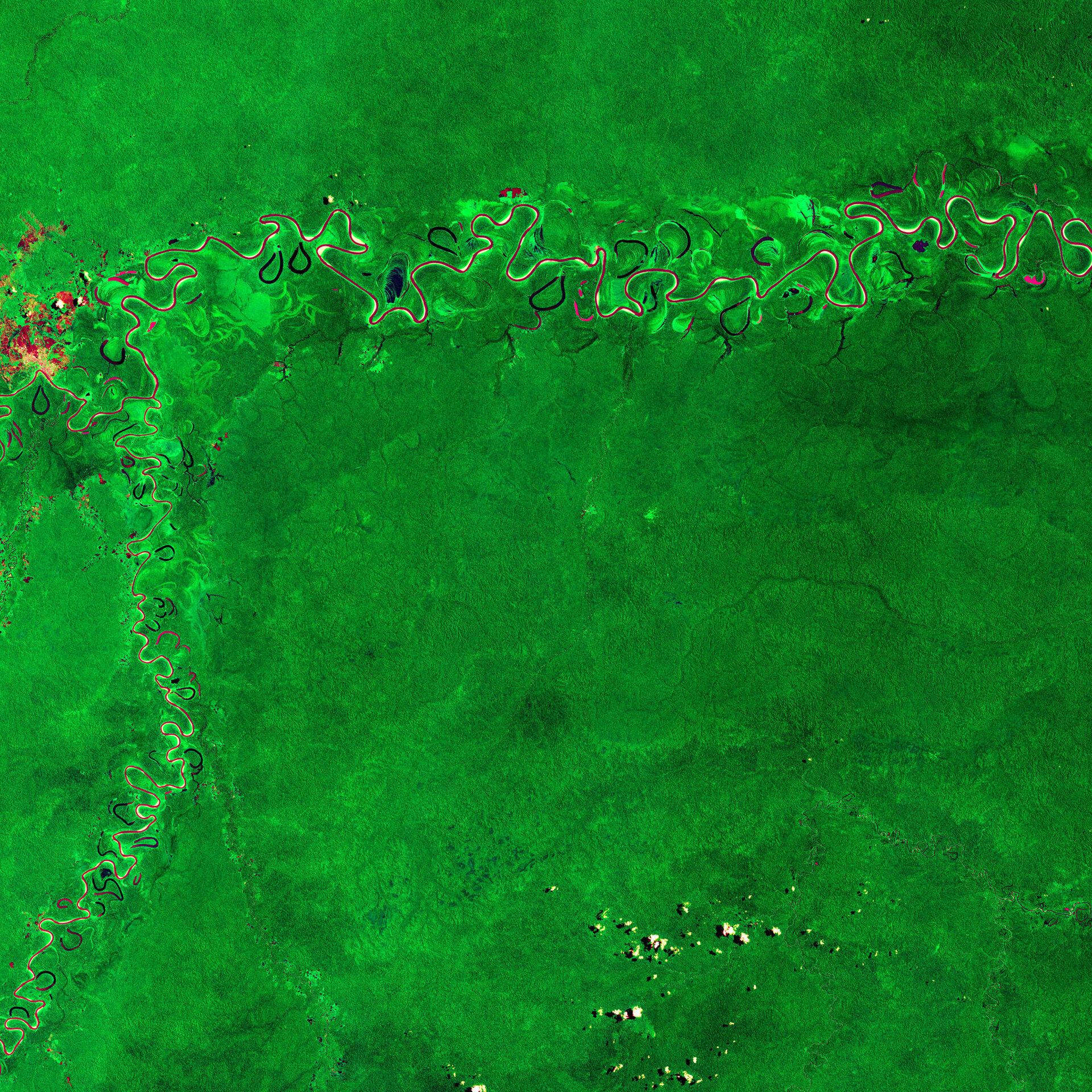The image is a predominantly green aerial or satellite view, capturing a possibly tropical area. The lush green background, which constitutes roughly 90-95% of the image, is interspersed with dark splotches. In the top portion of the image, a river-like channel of a different shade of green runs horizontally, contrasting with the main background. This channel contains white, blue, and red lines, suggesting the flow of water or other natural features. On the left side of the image, near the channel, there are red and orange splotches that add to the vibrant character of the scene. The channel curves and extends down toward the bottom left corner before exiting the frame. In the lower-right quadrant, small, irregularly shaped white dots, possibly resembling crumbs or light reflections, are scattered. The overall composition, with flowing water-like features and cloud-like formations, indicates a landscape captured from above, blending natural and possibly digital elements.